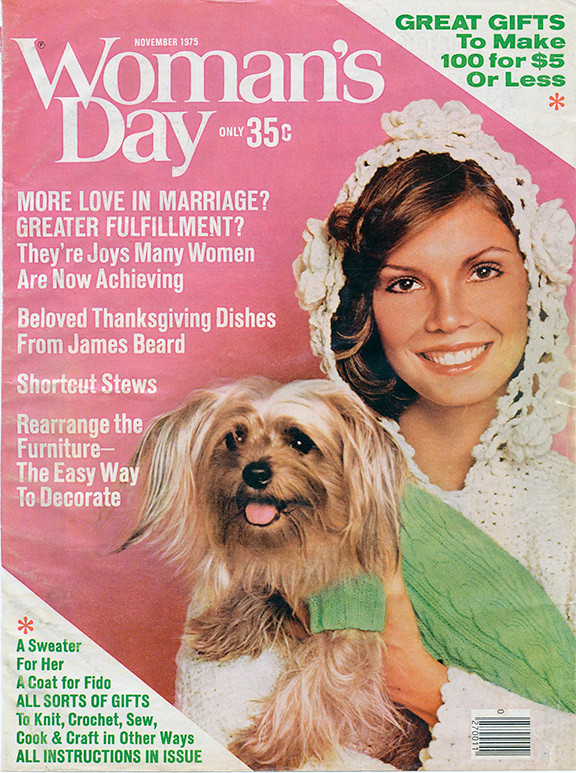This is a cover of an old November 1975 issue of Woman's Day magazine, priced at only 35 cents. The background is predominantly light pink, with white triangles in the top right and bottom left corners featuring additional text. In the top left corner, it reads "Woman's Day, only $0.35." Below that, the text elaborates on the issue's contents, including "More Love and Marriage, Greater Fulfillment, Their Joys Many Women Are Now Achieving," "Beloved Thanksgiving Dishes from James Beard," "Shortcut Stews," and "Rearrange the Furniture, The Easy Way to Decorate."

On the right half of the cover, a smiling woman with very white teeth and brown hair is depicted. She is dressed in a white lace or crocheted outfit, complete with a headpiece adorned with knitted flowers. She holds a small, brown and white dog wearing a green argyle sweater. 

Additionally, the top right corner announces, "Great gifts to make, 100 for $5 or less," while the bottom left corner highlights "A sweater for her, a coat for Fido, and all sorts of gifts to knit, crochet, sew, cook, and craft, with all instructions in the issue." All text on the magazine cover is printed in white letters.